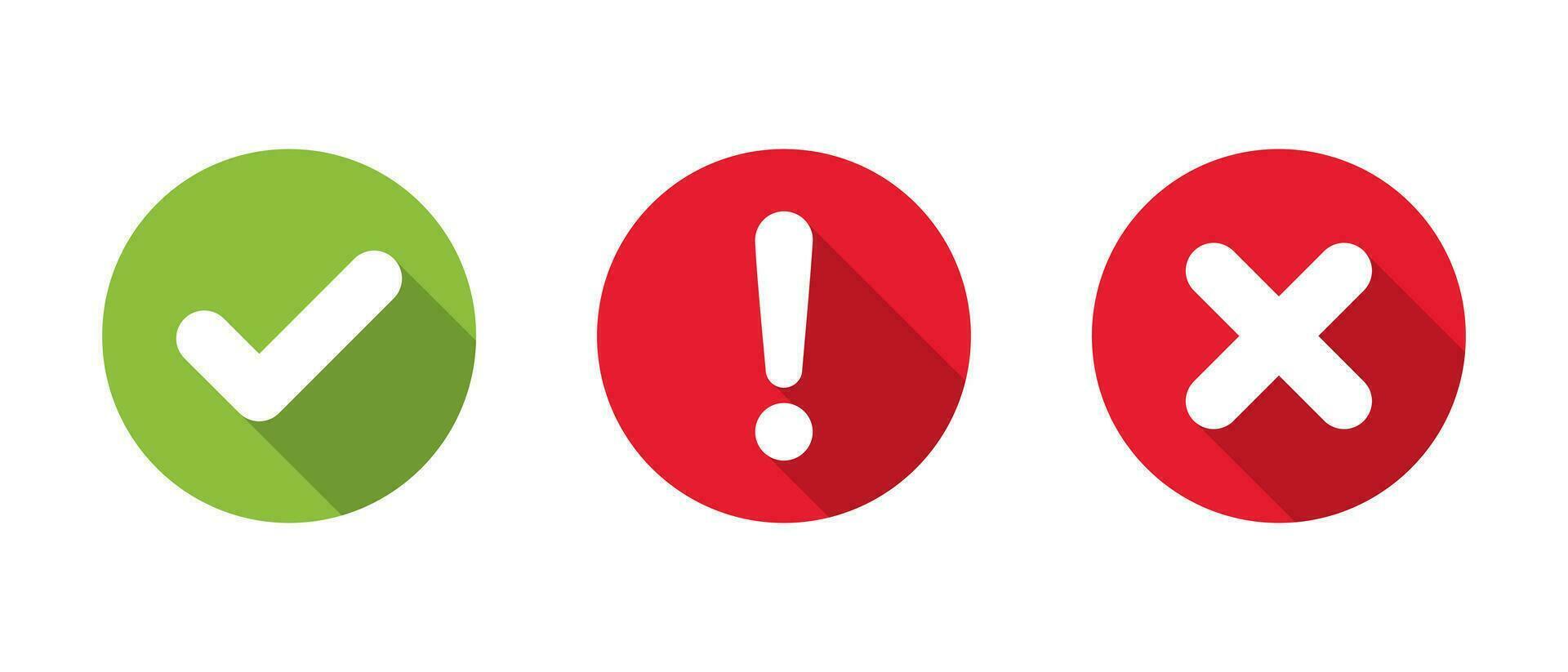The image features an illustration of three equally sized circles, centrally positioned against a completely white background. The leftmost circle is green, centered with a white check mark, while the middle circle is red, containing a white exclamation point. The rightmost circle is also red and displays a white X mark at its center. Each symbol casts a subtle shadow to the right, creating a slight darker gradient effect, as if illuminated by a light source from the left. The design is simple and consistent with modern web icons, often seen in digital and computer contexts, evoking a sense of caution or notification.